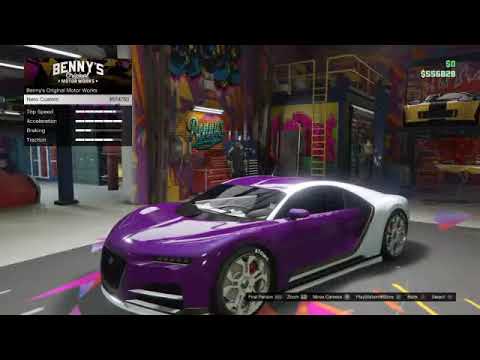The image portrays a detailed 3D-rendered scene from the popular video game GTA 5, depicting a car customization garage, specifically Benny's Original Motor Works. The focal point of the image is a compact, low-to-the-ground sports car with a sleek, aerodynamic design. Its front half is painted purple, transitioning to white towards the back. The car features large, black wheels and tinted windows. The garage's large, gray concrete floor and colorful walls, adorned with an explosion of neon graffiti in magenta and yellow, set a vibrant atmosphere. Visible in the background, another sports car is positioned on a lift. At the top left corner of the image, the text "Benny's" is prominently displayed, alongside blurry game statistics and currency information. The top right corner shows a dollar sign with an amount, currently reading $556,829. Various in-game options and prices are also visible, indicating this is the screen where players choose and customize their vehicles before racing.